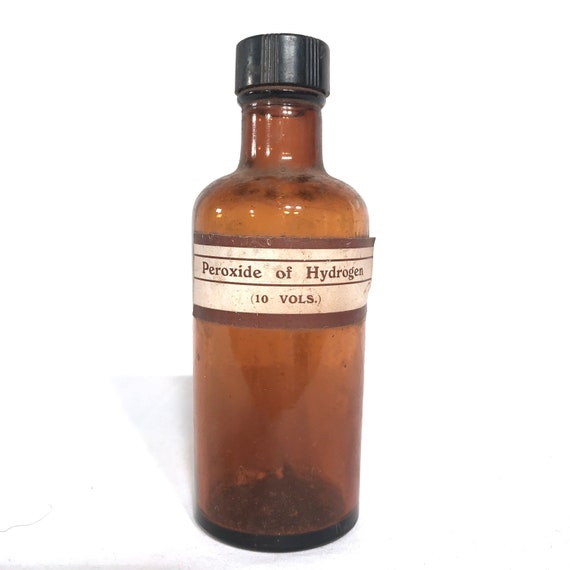The image depicts a vintage glass bottle labeled "Peroxide of Hydrogen, 10-VOLS," an old-fashioned term for hydrogen peroxide. The cylindrical bottle, made of brown glass, narrows at the neck and is sealed with a black plastic twist cap, suggesting it might be from the mid-20th century rather than the earlier 1900s. Notably, unlike contemporary plastic containers, this bottle has an archaic charm that evokes the 1940s or 50s era. The label itself, featuring brown text on a white background and appearing worn and partially peeling, adds to the antique aesthetic. The bottle is empty save for some possible residue at the bottom, and its transparent material, tinted brown, is reminiscent of old iodine bottles. This unique item stands out not only for its historical appearance but also for its deviation from modern packaging.